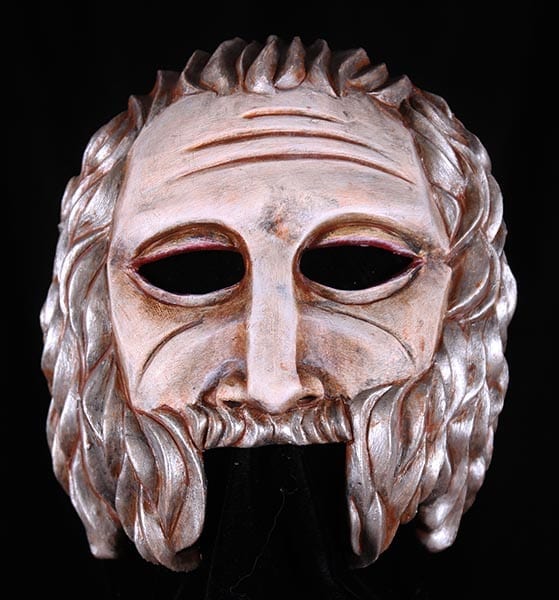The image features a metallic mask set against a complete dark black background. The mask portrays a masculine face with a distinctive, antiquated design suggestive of ancient use, possibly in battles or theatre. The face depicted has a long, straight nose leading to a prominent moustache and beard that connects seamlessly to wavy, silver hair encircling the head. The mask is detailed with three deep, progressively larger furrowed wrinkles on the forehead and additional wrinkled lines beneath large eye holes, meant for the wearer to see through. The mouth area of the mask is defined by a square cutout, leaving the wearer's mouth exposed. The overall coloration presents a striking contrast, with the face resembling a light tan or brownish tint, reminiscent of wood.